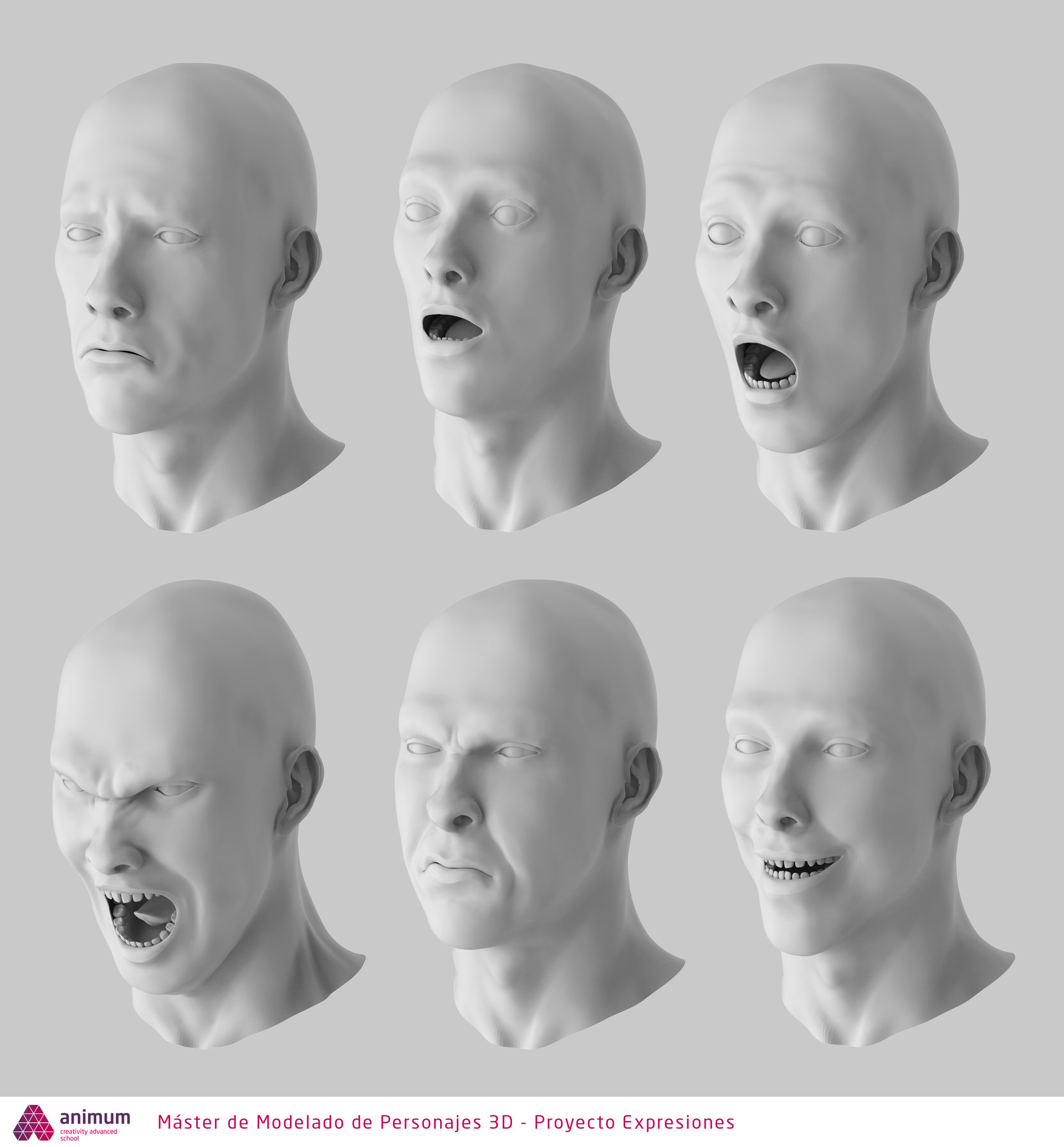The image showcases a set of six 3D-rendered, bald male heads, each displaying a distinct facial expression. Arranged in two rows of three, these models are entirely white, with no color differentiation. The top row features the following expressions: on the left, a frowning face; in the middle, an agape mouth suggesting shock or surprise; and on the right, a wider open mouth indicative of extreme surprise or horror. The bottom row continues with intense emotions: the leftmost head shows extreme anger or distress with a furrowed brow, the middle head has a look of disgust as though tasting something bitter, and the rightmost head presents an eerie, unnerving smile. Beneath the images, there is text reading "Animum Creativity Advanced School" along with "Master de Modelado de Personajes 3D Proyecto Expressions," denoting the institution and project responsible for these detailed 3D character models.